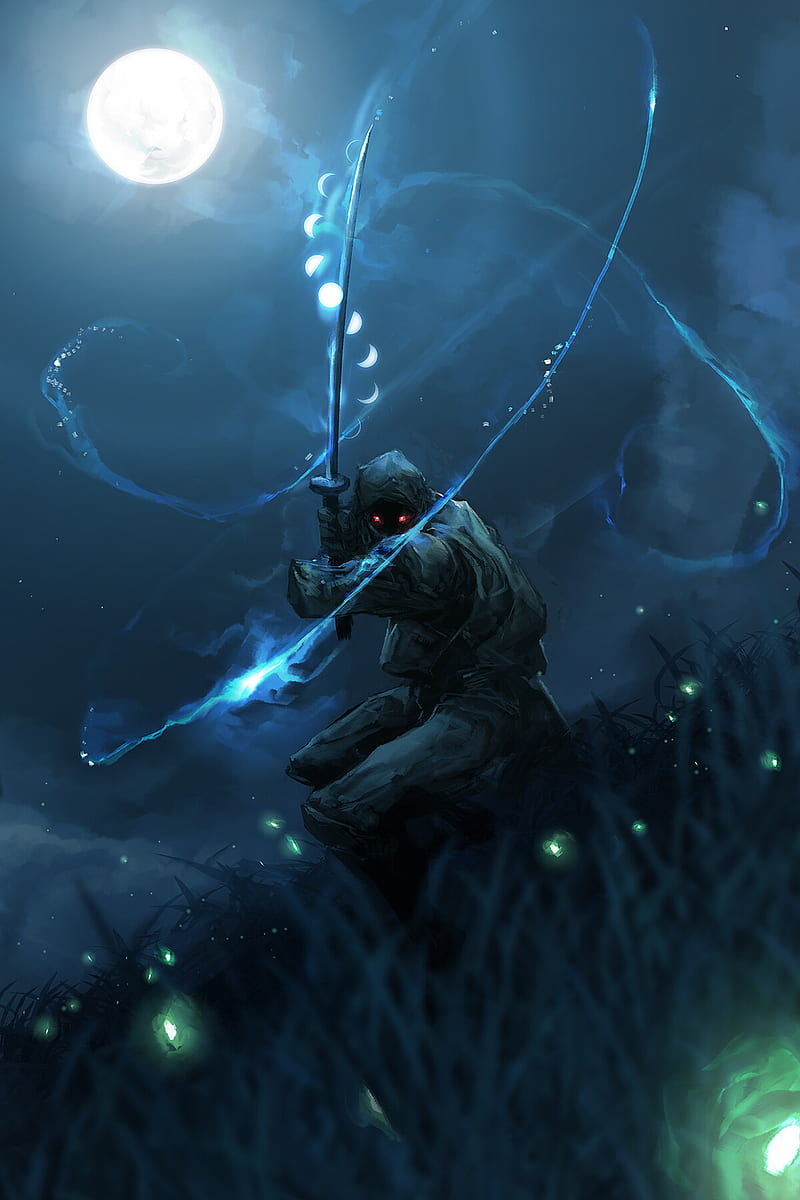This image depicts a highly detailed, computer-generated graphic, possibly reminiscent of artwork from a video game. In an outdoor setting illuminated solely by a glowing moon in the top left corner, a fearsome figure stands poised. The character, resembling a ninja or a menacing monster, is cloaked entirely in black, with only its piercing red eyes visible. This enigmatic figure wields a giant samurai sword, holding it upright as a swirling blue line illustrates the dynamic motion of the weapon. Smaller moon phases spiral around the sword, adding a mystical touch to the scene. In contrast, the bottom right corner reveals an image reminiscent of a cave ceiling with a distant light, while green splotches of light scatter across the ground. This captivating image, likely created digitally with a stylus, exudes a blend of dark, fantastical elements and exceptional graphical artistry.